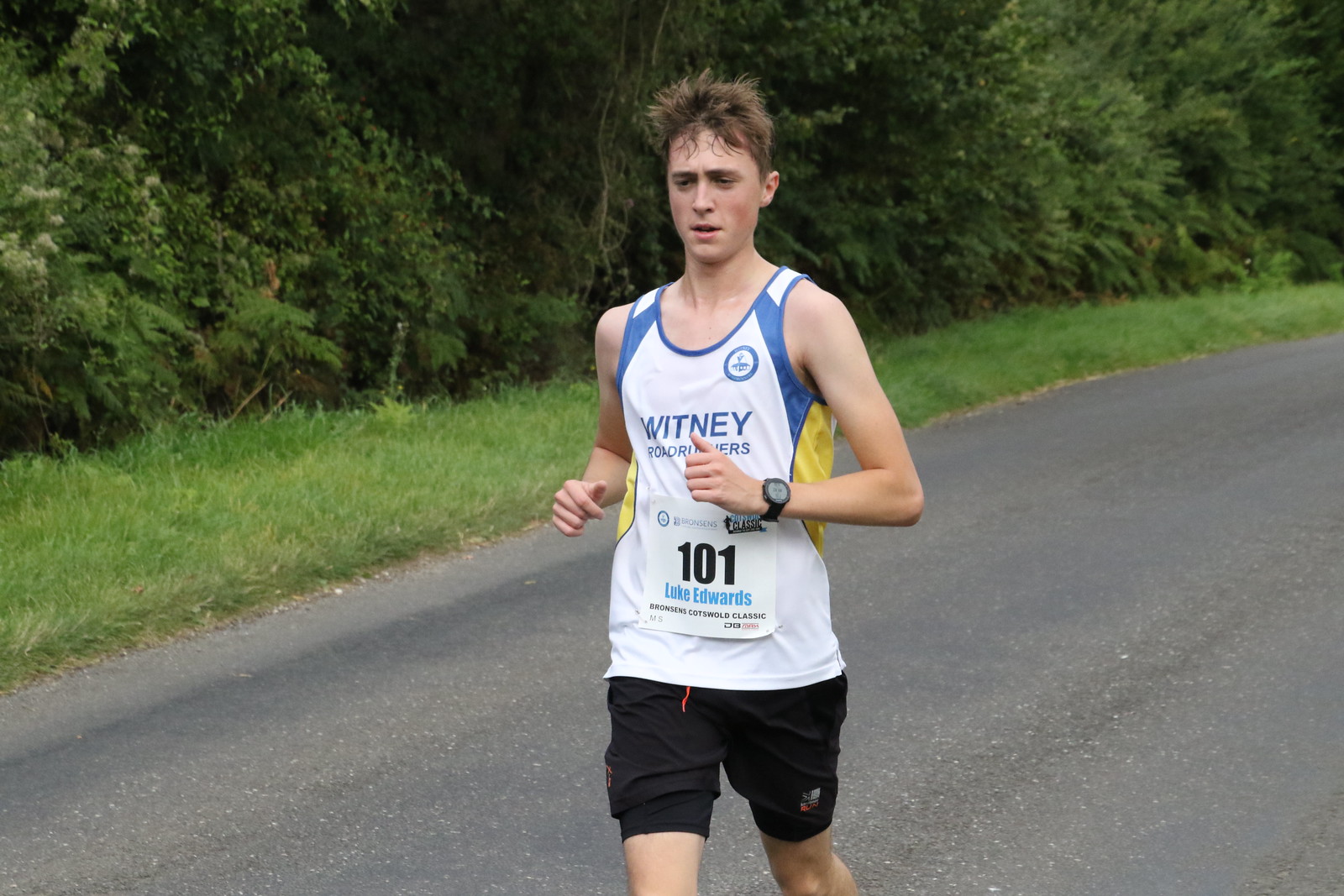A white man with brown hair, shorter on the sides and longer on the top, is running mid-stride on an unmarked paved road, surrounded by green grass, high bushes, and a tree line in the background. He is wearing a white tank top with blue and yellow accents that reads "Whitney Roadrunners," and black shorts. There is a number tag on his stomach that displays "101 Luke Edwards," indicating he is participating in a race. A black wristwatch adorns his wrist as he looks forward, with his hands held slightly out in front of him. The man appears to be in his 20s, and his lean physique is complemented by the sleeveless tank top, revealing his arms.